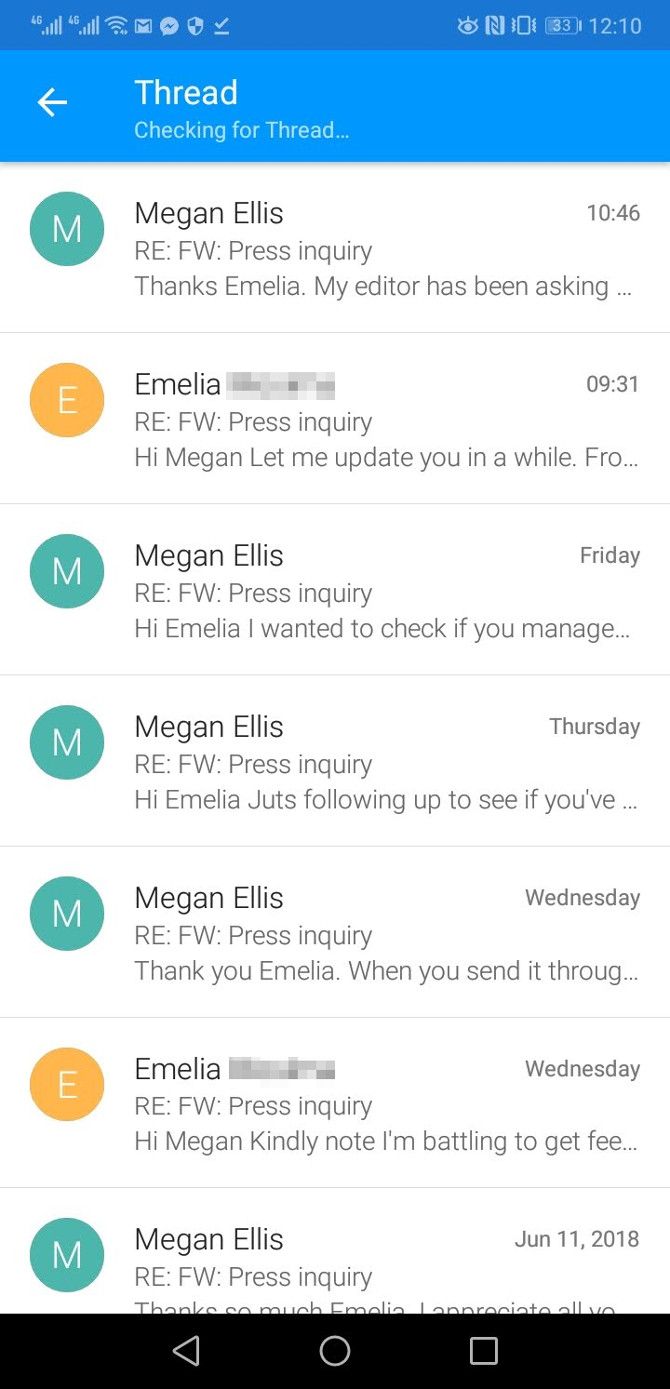This image is a screenshot taken in portrait mode, most likely from a phone. The screenshot is organized into a vertical column layout. The upper left-hand corner features a large blue stripe that stretches diagonally to the right-hand corner. In the top-right corner, the battery is at 33% and the time displayed is 12:10. 

Beneath this, there is a light blue row with a back arrow icon, followed by the text "Thread" and "Checking for Thread." Below this row, the screenshot reveals a series of emails. Each email is presented in an individual row, accompanied by the first letter of the sender's name in a colored block on the left-hand side.

The sequence of emails begins with:
- "M" in a green block, from Megan Ellis: "Press Inquiry - Thanks Amelia, my editor has been asking."
- "E" in an orange block, from Amelia: "Press Inquiry - Hi Megan, let me update you in a while."
- Megan Ellis again: "Hi Amelia, I want to check if you managed."
- Megan Ellis: "Hi Amelia, just following up to see if you've spelled wrong."
- Megan Ellis: "Thank you Amelia, when you send it through."
- Amelia: "Hi Megan, kindly note I'm battling to get fee."
- Megan Ellis: "Thanks so much, Amelia, I appreciate."

At the bottom right-hand corner of the screenshot, the date displayed is June 11, 2018. The email exchanges span several days, and timestamps visible above the email rows indicate days of the week, such as Wednesday, Thursday, and Friday, with times like 9:31 and 10:46. The emails' timestamps suggest that the current date is around Friday or Saturday, approximately June 15, 2018.